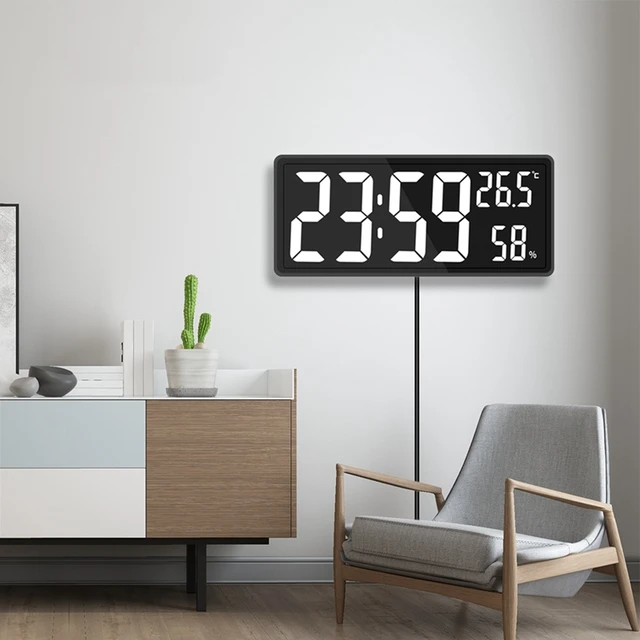This photograph captures a meticulously arranged contemporary living space with a blend of modern and retro elements. Central to the scene is a sleek armchair with a wooden frame and light grey cushioning, positioned against a pristine, white wall. Displayed prominently above the chair is a large digital clock featuring a black background and white digits, reading 23:59, with additional displays of 26.5 degrees Celsius and 58% humidity.

To the left of the chair, a stylish, low-profile console runs along the wall. The console is a tricolor unit with sections finished in brown, blue, and white, and is supported by sturdy black metal legs. Atop the console sits a white vase housing a cactus, flanked by a couple of distinct rocks and hints of a framed photo or artwork. Enhancing the room's modern aesthetic, the console's drawers—a blue top drawer and a white bottom drawer—remain closed, maintaining a clean, streamlined appearance.

The room is bathed in natural light that highlights the wooden flooring, adding warmth to the space. This carefully curated corner suggests a fusion of functionality and style, typical of a room designed for both relaxation and visual appeal.